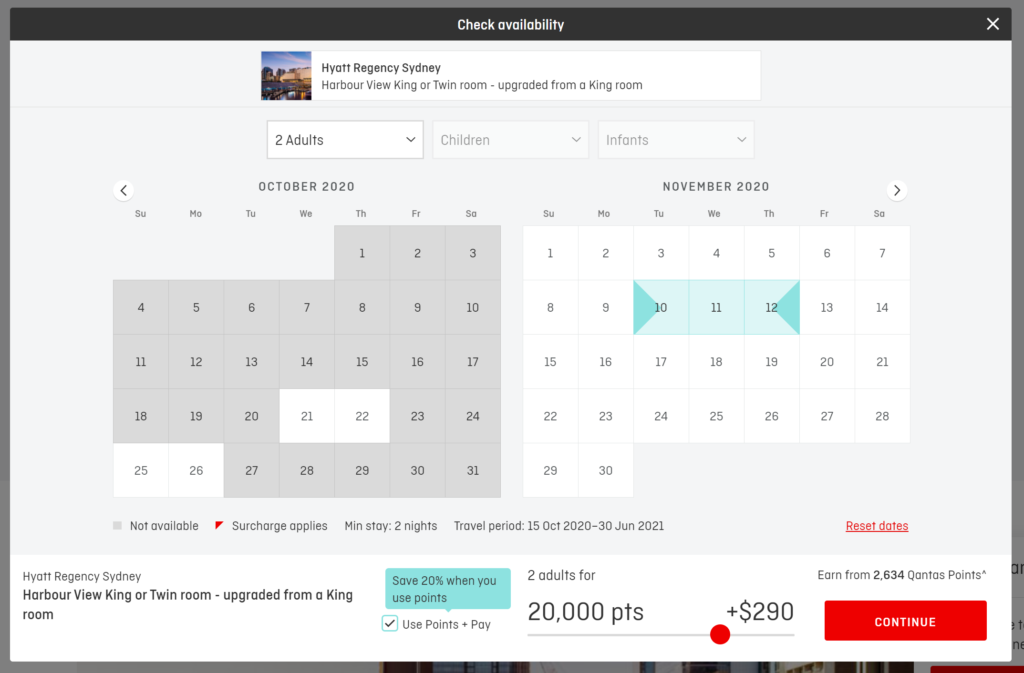The screenshot depicts the availability of rooms at the Hyatt Regency in Sydney for a booking. The interface features a pale grey background with three boxes under the banner indicating the presence of two adults, no children, and no infants. The calendar displays two months: October 2020 and November 2020. Dates from November 10th to the 12th are highlighted in green, suggesting a potential booking for those two nights.

Below the calendar, a legend explains the availability status, applicable surcharges, minimum stay requirements of two nights, and specifies the travel period must fall between October 15, 2020, and June 30, 2021. At the very bottom, a white banner details the room type: "Harbour View King or Twin Room upgraded from a King Room" and presents a special offer. Next to this, in black text on a green background, it mentions a 20% discount when using points, a promotion that has been selected.

The booking details are summarized: two adults for 20,000 points plus $290, with the additional benefit of earning 2,634 Qantas points. Finally, there is a red "continue" button for proceeding with the booking.